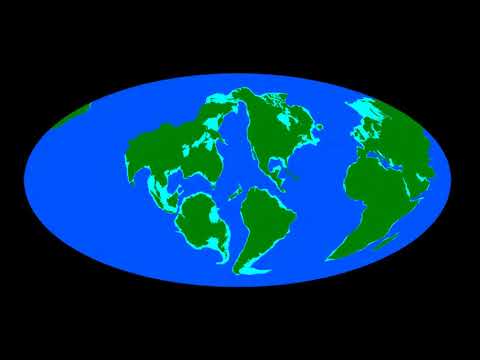This PNG-style image depicts a simplified, flattened projection of the Earth against a solid black background, accentuating a high-contrast view. The Earth, shaped more like an oval rather than a globe, features dark blue water and olive green landmasses. These landmasses include all seven continents: North America, South America, Europe, Asia, Africa, Australia, and a small part of Antarctica. Lighter teal hues trace the coastlines, and key inland waters, such as the Great Lakes, are highlighted in aqua blue. Displayed centrally without any textual annotations, the image focuses on a basic depiction, outlining the spatial relationship between continents without delving into intricate geographical details.